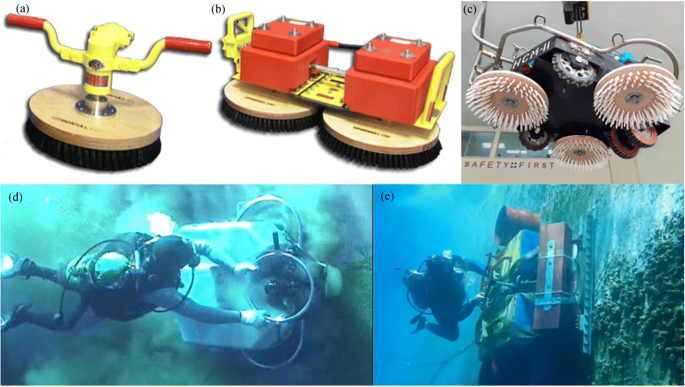The image is a detailed diagram divided into four sections, illustrating apparatus and their use in underwater scenarios. The top-left section, labeled "A," depicts a device with red handles on a yellow handlebar, mounted on a wooden disc with gray brushes beneath, reminiscent of bike handles. To its right, labeled "B," another apparatus features two orange cubes on a metallic yellow base, with tan circles and black brushes at the bottom. Directly beside it, labeled "C," is a device suspended from a ceiling-like structure with three tan wheels and white bristles, marked with the phrase "Safety First." 

The bottom-left section, labeled "D," shows a scuba diver in a black suit using a white apparatus against a rock formation in underwater surroundings. The diver's silver tank is clearly visible. The bottom-right section, labeled "E," illustrates another scuba diver interacting with a different but similarly structured yellow and red device. Both divers appear to be employing tools for cleaning or maintaining the ocean floor, indicating the multi-faceted utilities of these underwater apparatuses.